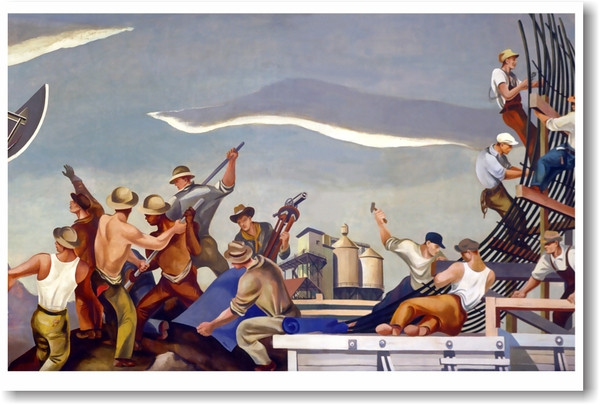In this detailed outdoor painting, a group of workmen is depicted engaging in various tasks against a predominantly gray sky, giving the scene an industrial, early 20th-century vibe. Men with brown hats, some shirtless, are scattered across the left side of the image, wielding shovels and appearing to dig into a mound of dirt while one individual holds a blue sheet-like material. On the right side, several men are seen working on a curved, metal-like structure composed of long beams, climbing and hammering with tools. The background features an industrial building with tank-like structures or silos, reinforcing the gritty, work-intensive atmosphere of the scene. The overall composition conveys a clear division of labor, with distinct groups focusing on either metalwork or excavation. The painting emphasizes the grueling nature of manual labor set in an early industrial era, characterized by its undefined faces and steel-blue hues.